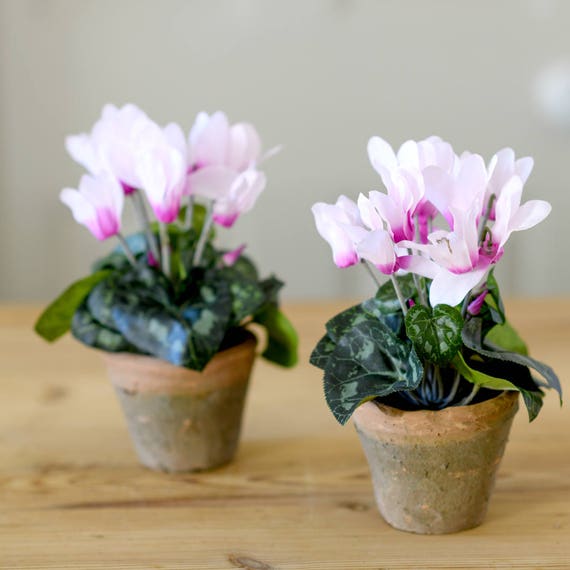This color photograph captures two small, identical potted plants sitting side by side on a wooden table with a subtle wood grain. The clay pots feature a lower section in green transitioning to a lighter clay color near the top, though one pot is slightly damaged and rough around the rim. Each pot is filled with glossy, well-maintained dark and light green patterned succulent leaves from which clusters of tulip-like flowers emerge. The flowers, in full bloom, exhibit slender, white petals with pink tinges pointing upward, and each bloom features a vibrant dark pink center. There are approximately six blooms per pot, all appearing healthy and vibrant. The plant on the right is in sharper focus and closer to the camera, while the plant on the left is slightly out of focus and positioned further back.